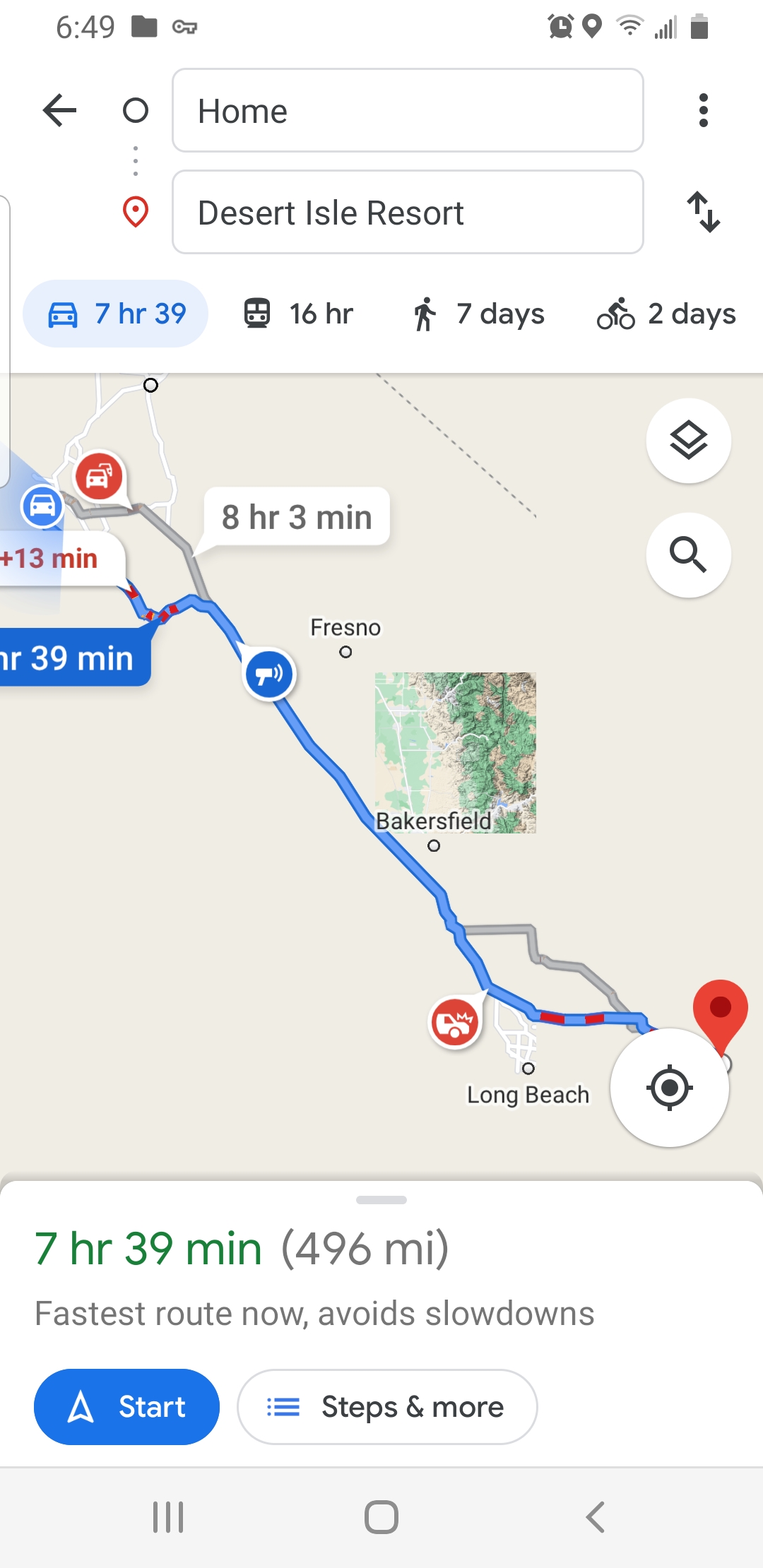The image showcases Google Maps navigation on a phone screen. In the status bar at the top, icons for the time (6:49), a folder, a key, an alarm clock, a marker arrow, Wi-Fi signal, cell data signal, and battery level are displayed. Below this, a search bar labeled "Home" is positioned above another labeled "Desert Isle Resort," marked with a red location pin.

Underneath the search bars, there are estimated travel times across different modes of transport: by car (7 hours 39 minutes), by train (16 hours), by walking (7 days), and by bicycling (2 days). The map below these estimates shows a route from the user's home to Desert Isle Resort, passing near Fresno and Bakersfield. The map is partially loaded, displaying only a small section.

The selected route is indicated with an estimated time of 7 hours and 39 minutes to cover a distance of 496 miles, marked as the fastest route while avoiding slowdowns. A secondary estimate indicates a travel time of 8 hours and 3 minutes, with a 13-minute delay noted. At the bottom of the screen, a green banner reaffirms the 7 hours and 39 minutes travel time, 496 miles distance, and the fastest route status. A blue button labeled "Start" invites the user to begin navigation, with options for "Steps & more" available.